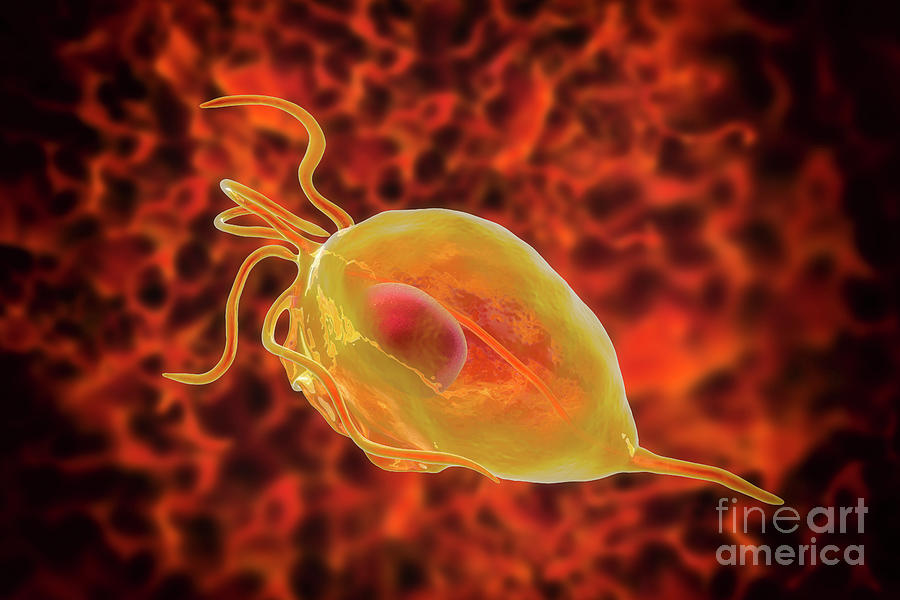This image appears to be an artistic rendering, potentially generated by computer or through digital art, of a single-celled organism, resembling an amoeba. The organism has a translucent yellow, almost lemon-yellow body with orange undertones, and it is characterized by several tentacle-like extensions protruding from its back and one from its front, which likely suggest motion or the way it swims. A pinkish-reddish nucleus is visible at its center, encased within a membranous structure. The transparent nature of the organism allows glimpses of the vibrant orange coloration behind it. The background features a visually striking, abstract design resembling a red and orange celestial explosion or fiery fog, lending a sense of heat and movement. The image includes the logo "Fine Art America" in the bottom right corner, confirming its nature as an art piece rather than a literal scientific photograph.